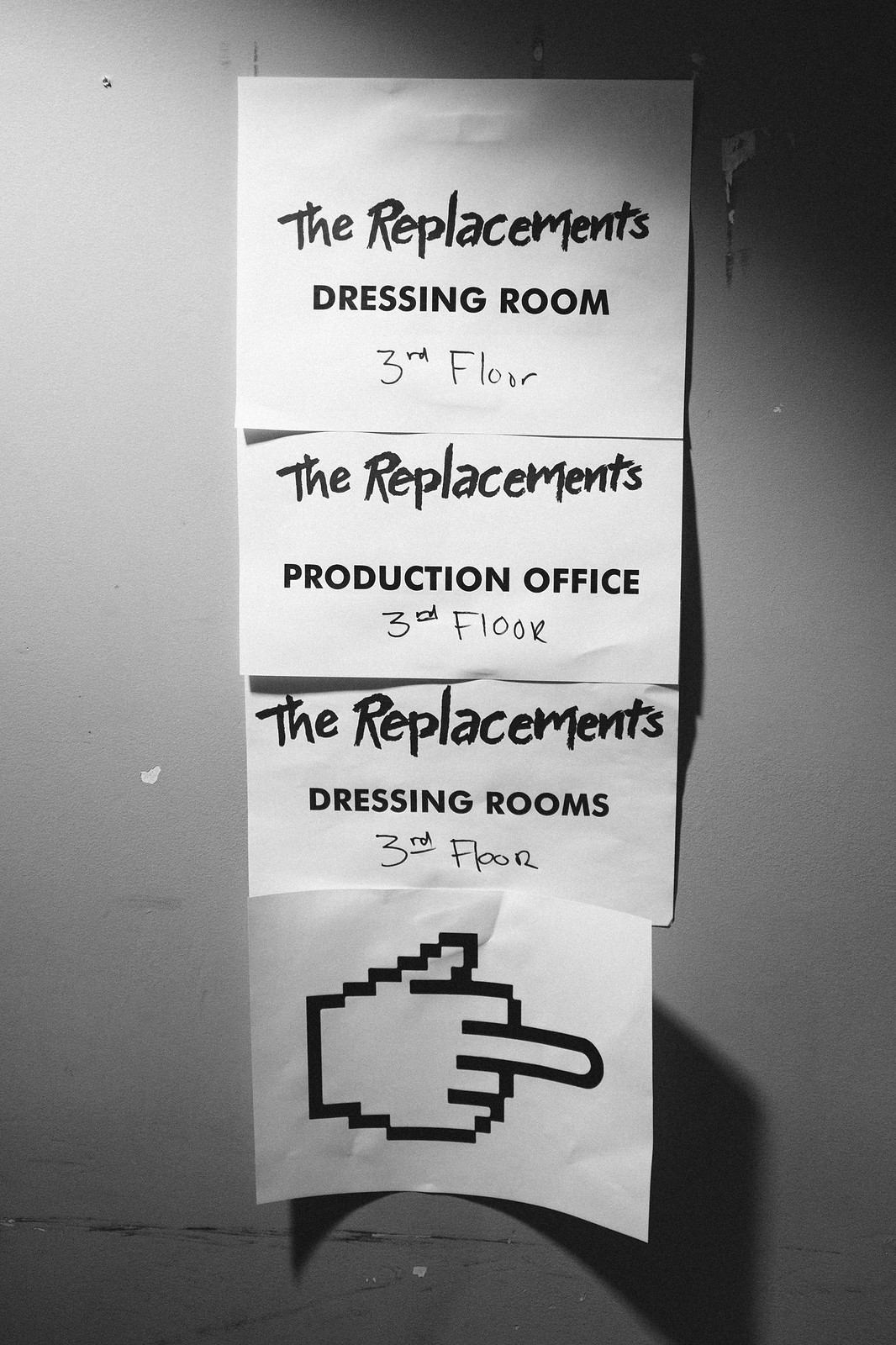The image depicts four square white pieces of paper that have been tacked to a gray wall, which bears visible dings and scrapes, indicating heavy use. Each paper, appearing to be in sequence, provides directions related to 'The Replacements.' The top sheet, in an action-oriented, possibly band-inspired font, reads "The Replacements Dressing Room," with the handwritten note, "3rd Floor." Below it, the second sheet states, "The Replacements Production Office," again noting "3rd Floor" in handwritten style. The third paper echoes the top, "The Replacements Dressing Rooms," with an underlined "3rd Floor" handwritten. The final paper features a computer-generated image of a pointing hand, notably using the middle finger, directing to the right. There is also residual evidence of previous papers on the wall, with torn white remnants sticking to the right side. The composition and style suggest a punk rock aesthetic, possibly connected to the band 'The Replacements.'